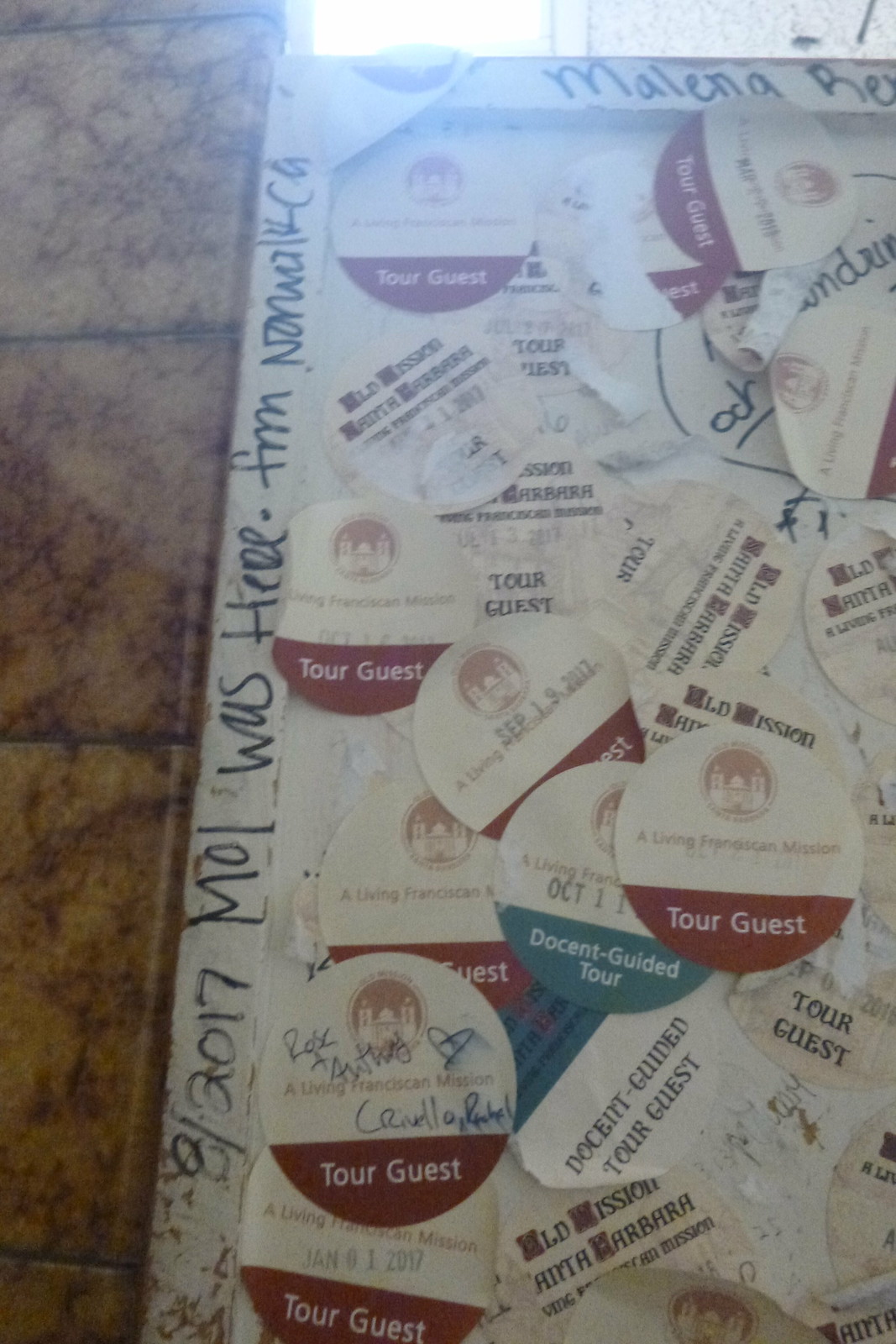This image features a visitor's board, possibly mounted against a wall or lying flat on a tile floor, capturing a collection of experiences from various guests. The primary attraction is a wooden-framed piece, behind glass or painstakingly glued directly onto the surface. The board is densely covered with numerous circular stickers, each denoting "tour guest" or "docent guided tour," many of which bear signatures or names. These stickers are layered so densely that reading individual ones is nearly impossible. Along the left border, a message scrawled with a black marker reads, "8-2017 Mel was here from Norwalk," with slight variations in the name, such as "Mole" or "Melina" appearing at different points. The board's surrounding area appears slightly dirty, hinting at a well-trodden part of the venue, possibly indicating it’s a spot where guests add their tour memorabilia after completing their visit.